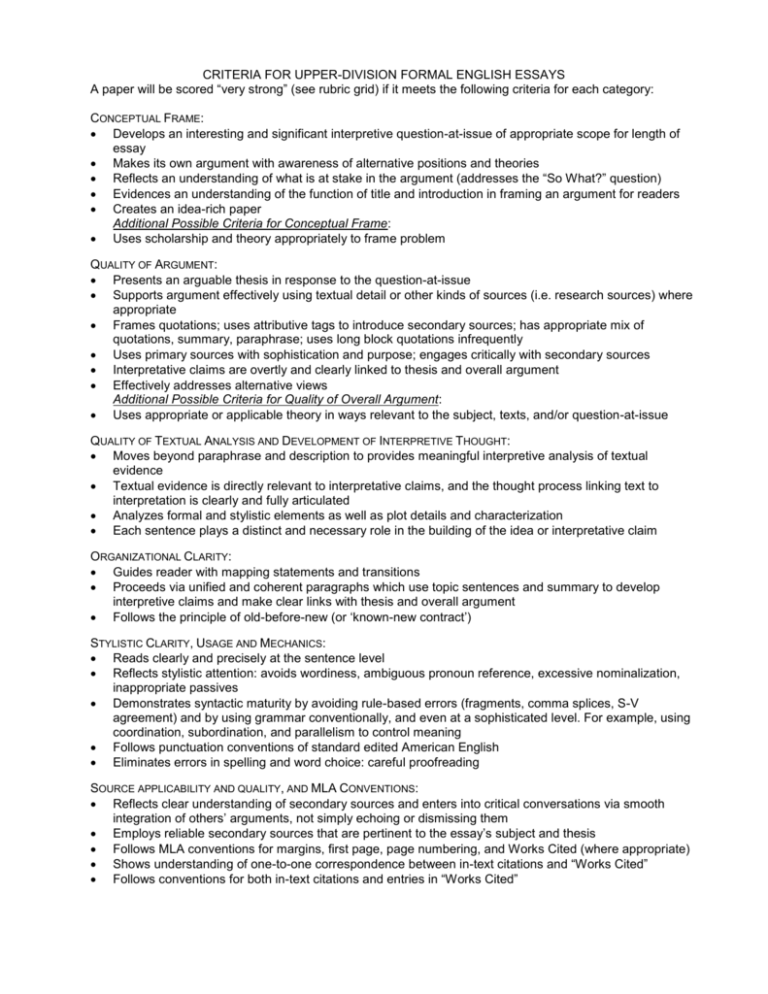This image depicts an extensive rubric for assessing upper-division formal English essays, featuring a structured list of criteria categorized into various sections. At the top of the page, the heading "Conceptual Frame" introduces six detailed bullet points. The next section, "Quality of Argument," elaborates with seven bullet points. Following that, "Quality of Textual Analysis and Development of Interpretive Thought" includes four bullet points. The "Organizational Clarity" category encompasses three bullet points. The "Stylistic Clarity, Usage, and Mechanics" section provides five bullet points. Finally, at the bottom, the "Source Applicability and Quality and MLA Conventions" cluster features an additional five bullet points. Notably, an underlined bullet point within the "Conceptual Frame" section highlights the criterion "Uses scholarship and theory appropriately to frame problem," suggesting added emphasis on this particular standard.